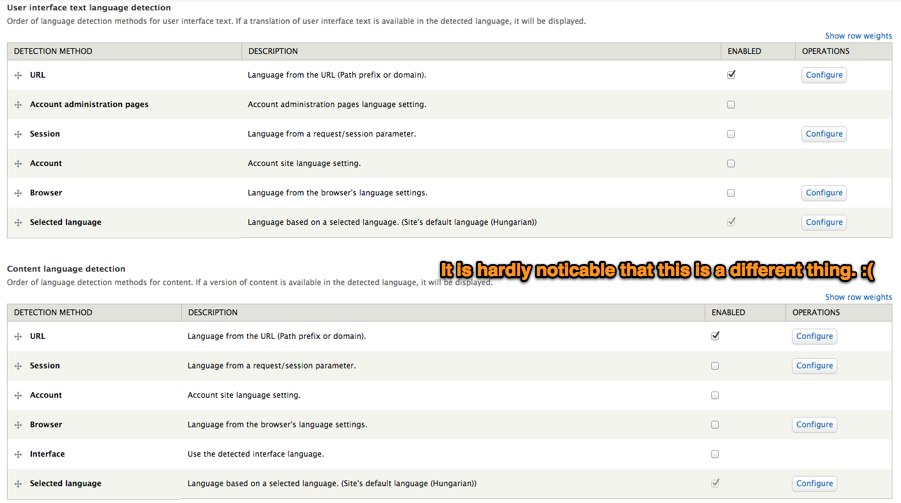This screenshot, seemingly from an interface configuration tool, illustrates the settings for language detection methods applied to user interface text. At the top of the screenshot, the title reads, "User Interface Text Language Detection: Order of Language Detection Methods for User Interface Text." 

The section specifies that if a translation of the user interface text is available in the detected language, it will be displayed according to the established order. Below this, a table is present with several columns labeled: "Detection Method," "Description," "Enabled," "Operations," "Show Row Weights," and "URL."

1. The first method listed is "Language from the User Path Prefix or Domain" with the "Enabled" box checked, followed by a "Configure" option.
2. Next, "Account Administration Pages Language Setting" is presented, indicating that the setting is enabled at the account administration page level, followed by "Session."
3. The "Language from a Request" method via the "Session Parameter" comes next with a "Configure" button beside it.
4. Then, "Account Site Language Setting" details how language from user accounts are specified.
5. Another entry is "Browser," which references the "Language from the Browser's Language Settings," also with the "Configure" option.
6. "Selected Language" shows language detection based on a user-selected language preference.
7. The "Site's Default Language" is indicated as Hungarian, with a checkbox marked, also having the "Configure" button.

Beneath this, a heading in orange highlights user-generated commentary: "It is hardly noticeable that this is a different thing," along with a sad face emoticon. The comment emphasizes the repetitiveness as the subsequent content mirrors the earlier details under the "Content Language Detection: Order of Language Detection Methods for Content." The secondary section similarly outlines that if content is available in the detected language, it will display accordingly, reiterating the same user interface language detection settings.

Overall, the individual's comment draws attention to the apparent redundancy and minimal clarity distinguishing between the sections, suggesting a need for clearer differentiation.